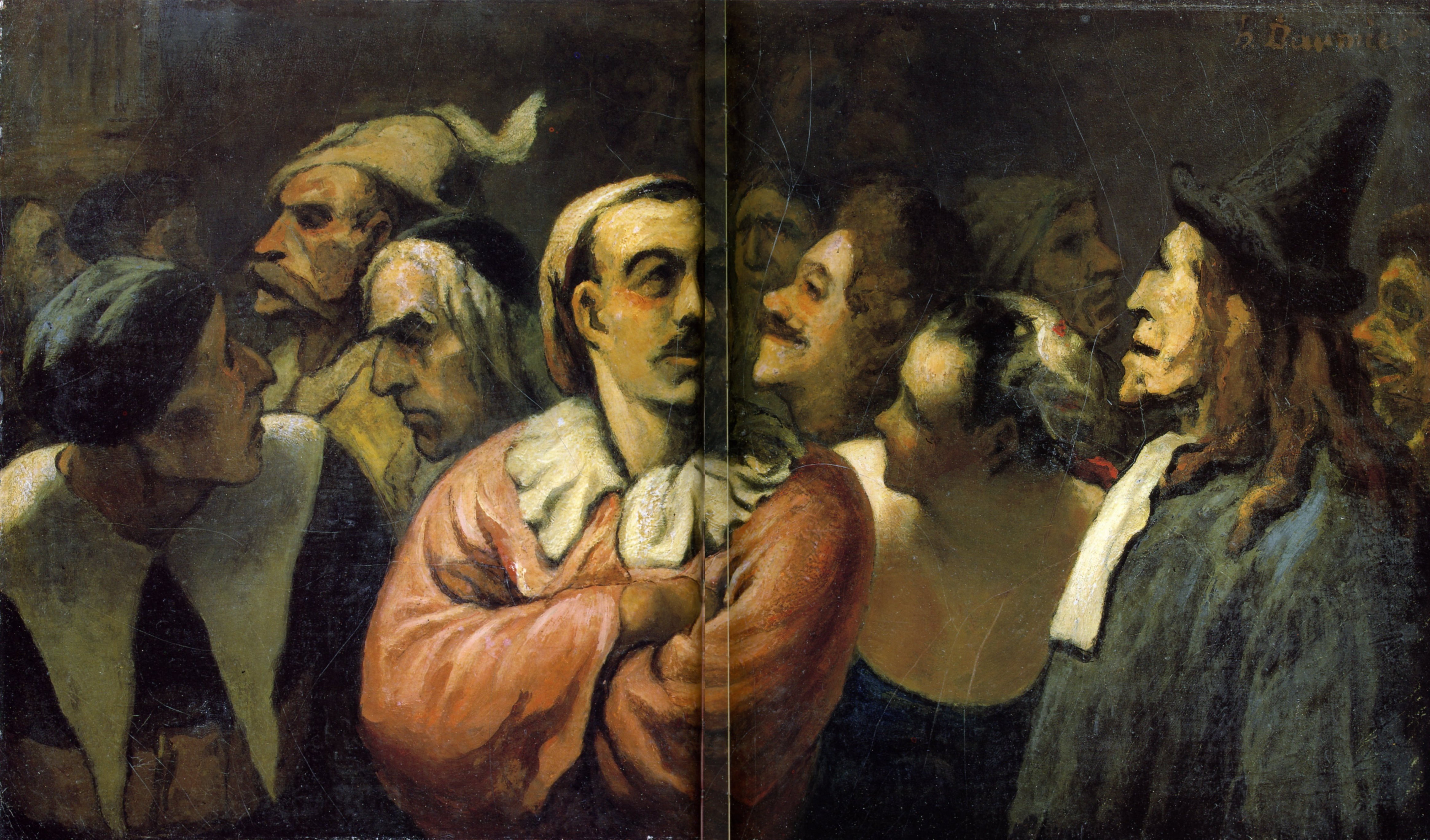The image is an old painting depicting a group of men, possibly important figures, in a somewhat Renaissance-style, realistic yet with an impressionist feel. The colors used are quite diverse, ranging from pink, dark green, blue, black, brown, and beige to various shades of gray, darker pink, and red. The setting displays these figures with the background featuring a muddy brown tone, and the characters themselves rendered in a neutral and muted palette, emphasizing grays, blacks, and tans.

At the center of the painting is a man dressed in a striking red cloak with a large billowing white collar, rosy cheeks, and his hair pulled back with a white cap. He has his arms folded around his middle and is looking to the right. To his left stands another man, also in a black robe with a large white collar, peering curiously at him. Further left, there appears to be a figure that might be a maid or chef, wearing black and white attire and a hairnet. Immediately behind her is a grumpy-looking man in soldier gear.

On the right side of the central figure, a man in a long black robe with a white collar and a pointed black hat stares intently at the man in red. The background is populated with many more, albeit lighter and more blurred figures, consisting predominantly of men. This creates the impression of a larger crowd, contributing to the painting's dense and rich composition.